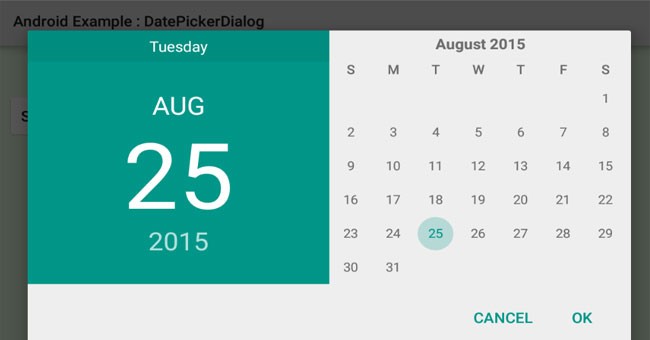The image depicts a calendar interface embedded within a software environment. The top, left, and right edges of the calendar are outlined in a dark gray or black border, suggesting that it is an overlay on another application screen. The background at the top of the image displays the title "Android Example: Date Picker Dialogue," written with camel case (DatePickerDialogue) formatting.

At the top center of the calendar is a green square with the day "Tuesday" written in white text. Below this header, a horizontal line separates the day of the week from the main calendar grid. The calendar shows the month of August 2015, labeled "AUG 25, 2015" in a prominent style. The days of the week (Sunday through Saturday) are abbreviated as SMTWTFS along the top of the calendar grid.

August 2015 is displayed with each date in black text, except for the 25th, which is highlighted with a light teal jade circle around it. At the bottom of the calendar, options to "Cancel" or "OK" are provided for user interaction. Overall, the interface is designed to allow users to select a specific date within the month of August 2015.